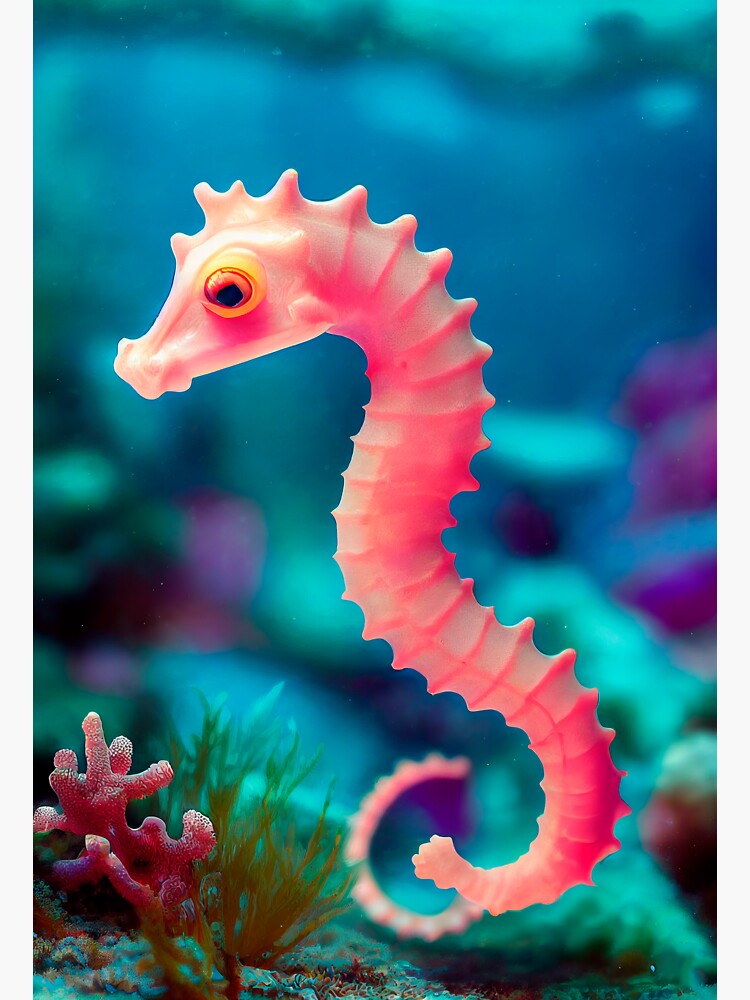In this photograph, a bright pink baby seahorse with an S-shaped, curling body and ridges along its sides and head appears to be swimming in a colorful underwater scene. The seahorse’s horse-like face features large pink eyes ringed with yellow, adding a striking contrast. Positioned in front of the seahorse are vibrant red corals and small green plants, enhancing the lively appearance of the underwater habitat. To the left, a piece of purple coral is visible, complemented by patches of green seagrass or seaweed. The background is intentionally blurred, showcasing a gradient of medium blue hues with hints of purple and green, and possibly the surface of the water at the very top of the image. While the photograph’s vivid and possibly digitally enhanced colors create an almost surreal appearance, it captures the enchanting and vivid beauty typical of tropical marine life.